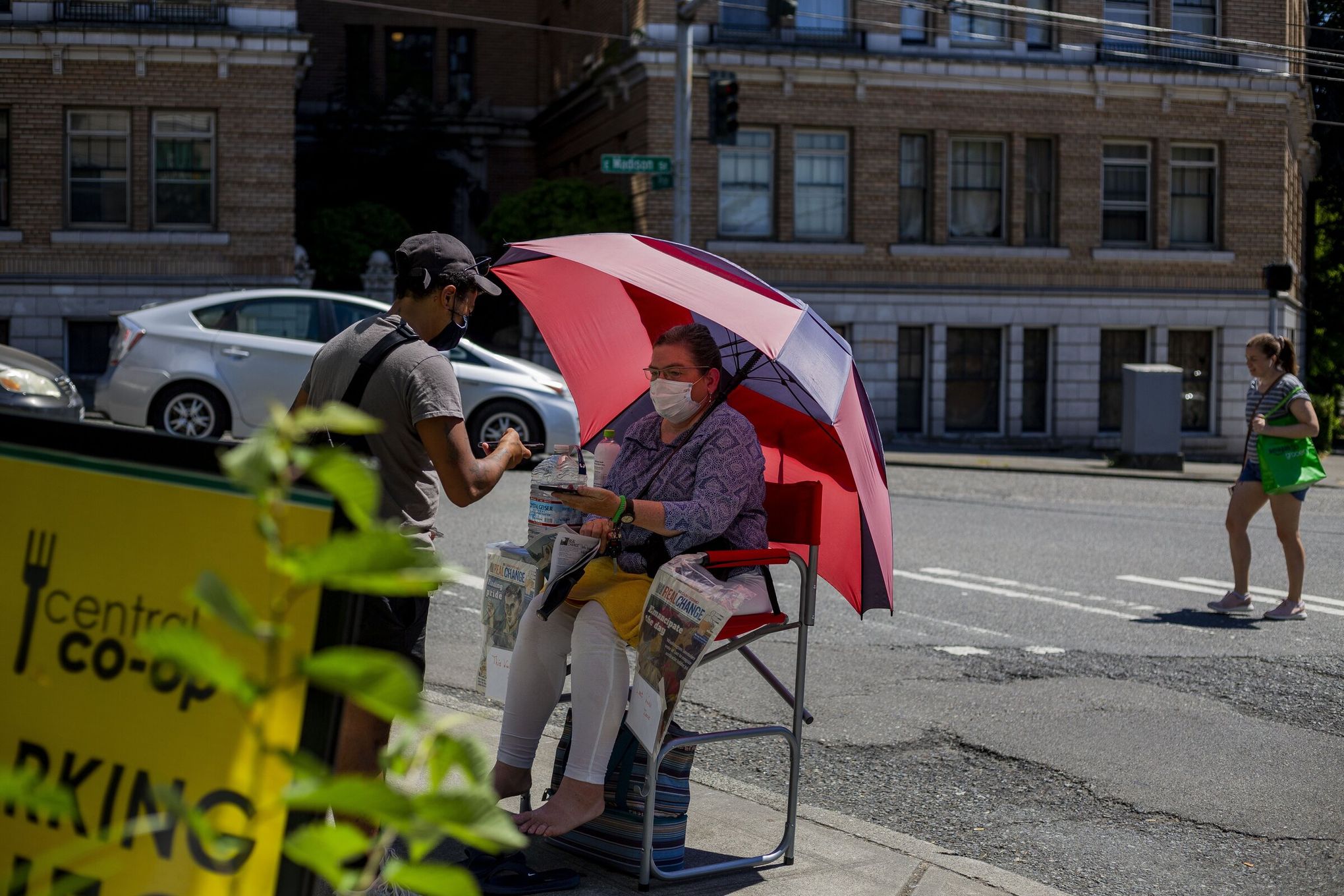The photograph, taken outdoors on a sunny day using natural light, appears to be a recent full-color square image of a busy city street scene. Dominating the top part of the image are a couple of brick buildings at least three stories tall. In the middle-right, a young woman is crossing the street from right to left. She is wearing a blue and white striped shirt, shorts, headphones, and carries a green bag. 

At the bottom left corner of the image, there is a yellow sign with black text hinting at "central co-op parking." Beside this sign, partially obscured by some plants, is a man in a gray t-shirt and dark shorts, with a black strap over his shoulder, who appears to be looking at something on his phone. 

Adjacent to him on the left sidewalk area, a woman is seated in a high metal chair with red arms and back. She is barefoot and wears white pants, a purple sweater, and a white COVID mask. With short gray hair and glasses, the woman shields herself from the sun using a large umbrella with pink, red, and white stripes. On one side of her, she has a large water bottle and several newspapers or magazines, suggesting she might be selling them. 

Across the bottom of the scene, cars travel from left to right along the street, further enhancing the city ambiance of this detailed and dynamic image.